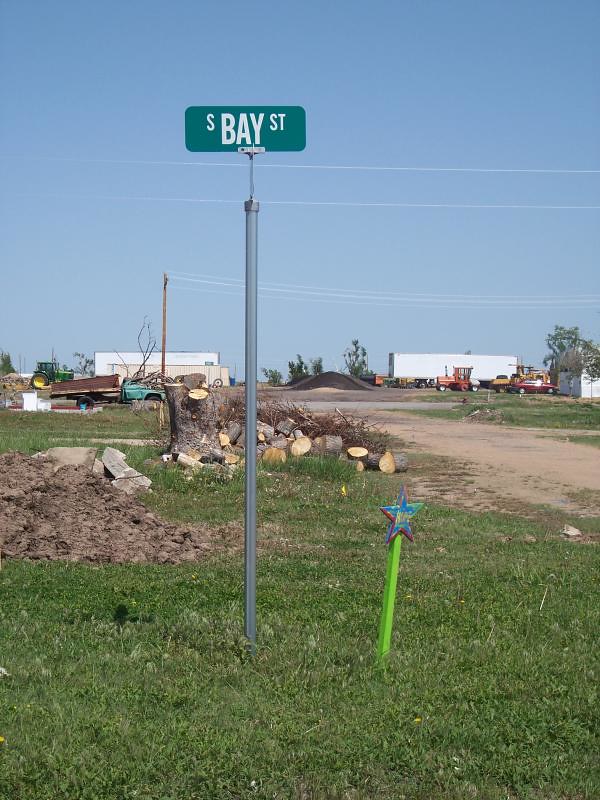In the photograph, we see a solitary street sign bearing the label "S Bay Street" or "South Bay Street" in white lettering atop a tall silver metal pole. The sign stands incongruously in a rural, somewhat desolate area characterized by dirt paths and grassy expanses, with no proper pavement in sight. Directly next to the sign, a small green pole adorned with a blue and green star, likely placed there by a child, adds a touch of whimsy.

The immediate surroundings include scattered piles of chopped logs, possibly intended for firewood, and a few rocks dotting the ground. Farther in the background, one can spot tractors and potentially some construction or warehouse-like buildings, suggesting a mix of agricultural and industrial elements. This area, devoid of any bustling activity or dense population, projects a quiet, rural ambiance with hints of ongoing or future development.